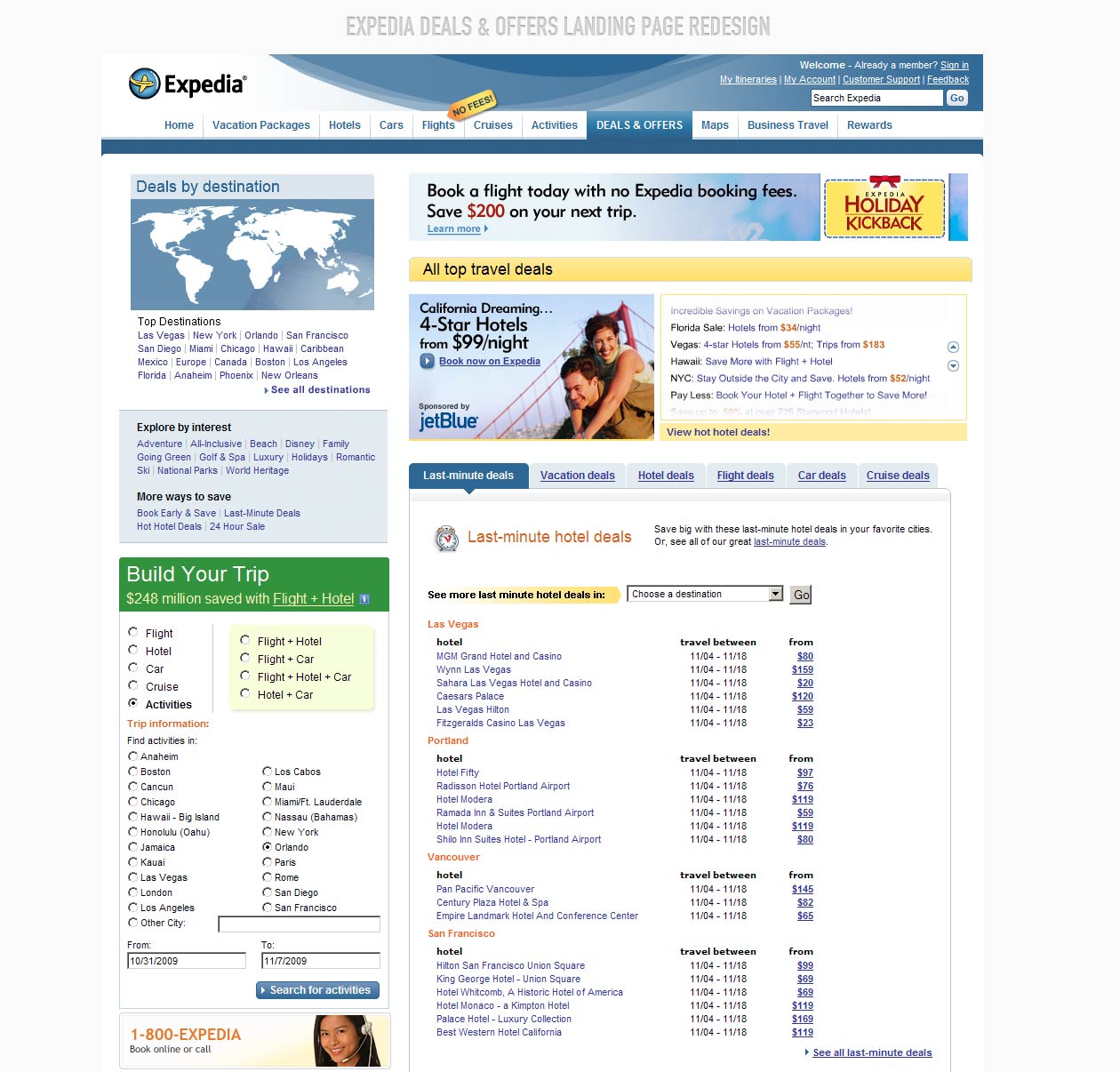This screenshot captures a detailed view of the Expedia website, prominently showing the "Deals and Offers" landing page. In the top left corner, the Expedia branding is evident with its name and recognizable circular logo featuring an airplane. At the top of the page, a navigation menu includes options for "Home," "Vacation Packages," "Hotels," "Cars," "Flights," "Cruises," "Activities," "Deals and Offers" (highlighted in this view), "Maps," "Business Travel," and "Rewards". 

To the right of the menu, there's a search box that allows users to find specific content on the Expedia site. The left sidebar offers a variety of deals based on destination and interest, listing options like early bookings, last-minute deals, hot hotel deals, and 24-hour sales. Below this is an interactive "Build Your Trip" section, where visitors can customize their travel plans by selecting combinations of flight, hotel, car, and activities. Standard city options are provided along with a field to enter a custom destination, as well as a contact phone number for Expedia's support.

On the right side of the page, there's a prominent "Book a Flight Today" section, displaying current savings and deals. Highlighted deals include special hotel rates in California through JetBlue, alongside various other promotional offers. Last-minute deals are featured with a dedicated section showing discounted hotel options in cities such as Vancouver, Portland, Las Vegas, and San Francisco, complete with available travel dates and special rates.